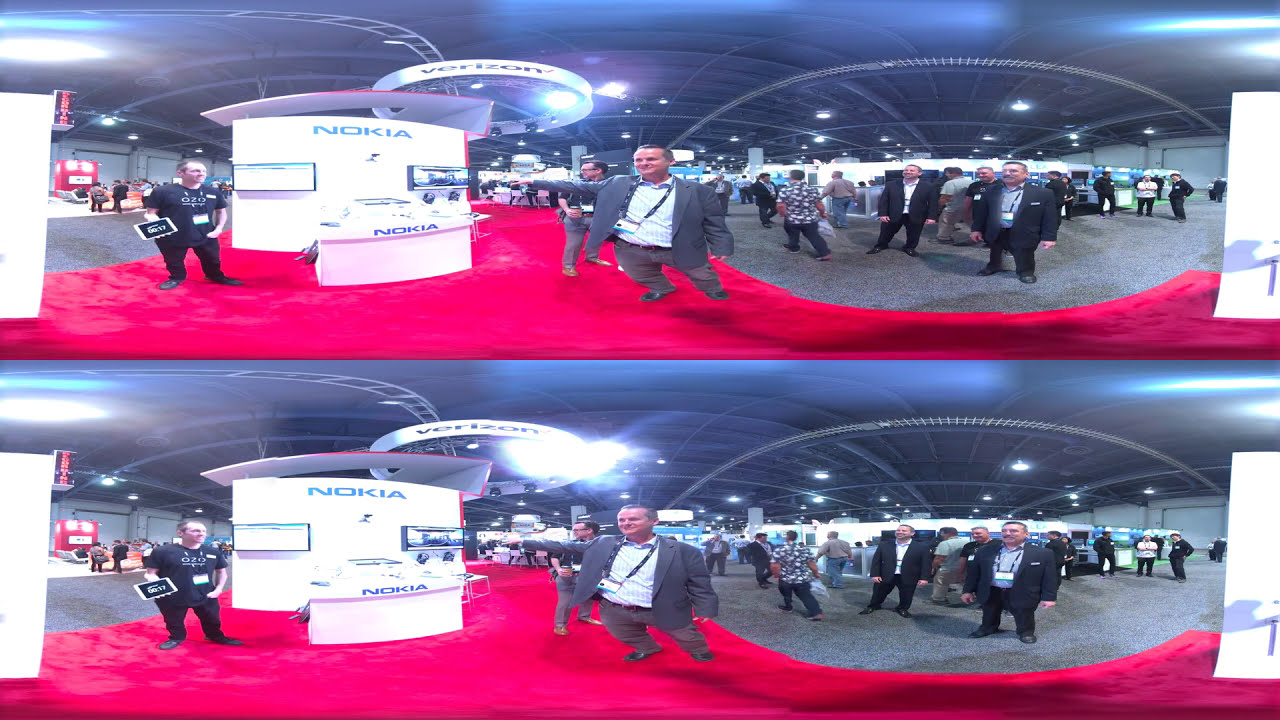The image depicts a panoramic, distorted 360-degree view with a fisheye effect, where the same photo is repeated on the top and bottom halves of the frame. At the heart of a bustling electronics expo, a man in a gray suit stands centrally, wearing a lanyard that signifies his participation in the event. The setting is a large, industrial-like hall with towering ceilings, partially visible walls, and a red carpeted floor. Around him, numerous attendees, primarily middle-aged and dressed in business attire, are milling about.

To the left of the image, a prominent booth displays the name "Nokia" twice, once on the front table and again on a sign behind it. At this booth, a person dressed in black holds a tablet, appearing ready to engage with visitors. In the background, additional signage for Verizon can be seen, further suggesting the expo’s technological focus. The overall scene is dynamic, filled with people smiling, conversing, and exploring various exhibits, capturing the energetic atmosphere of a high-profile tech convention.